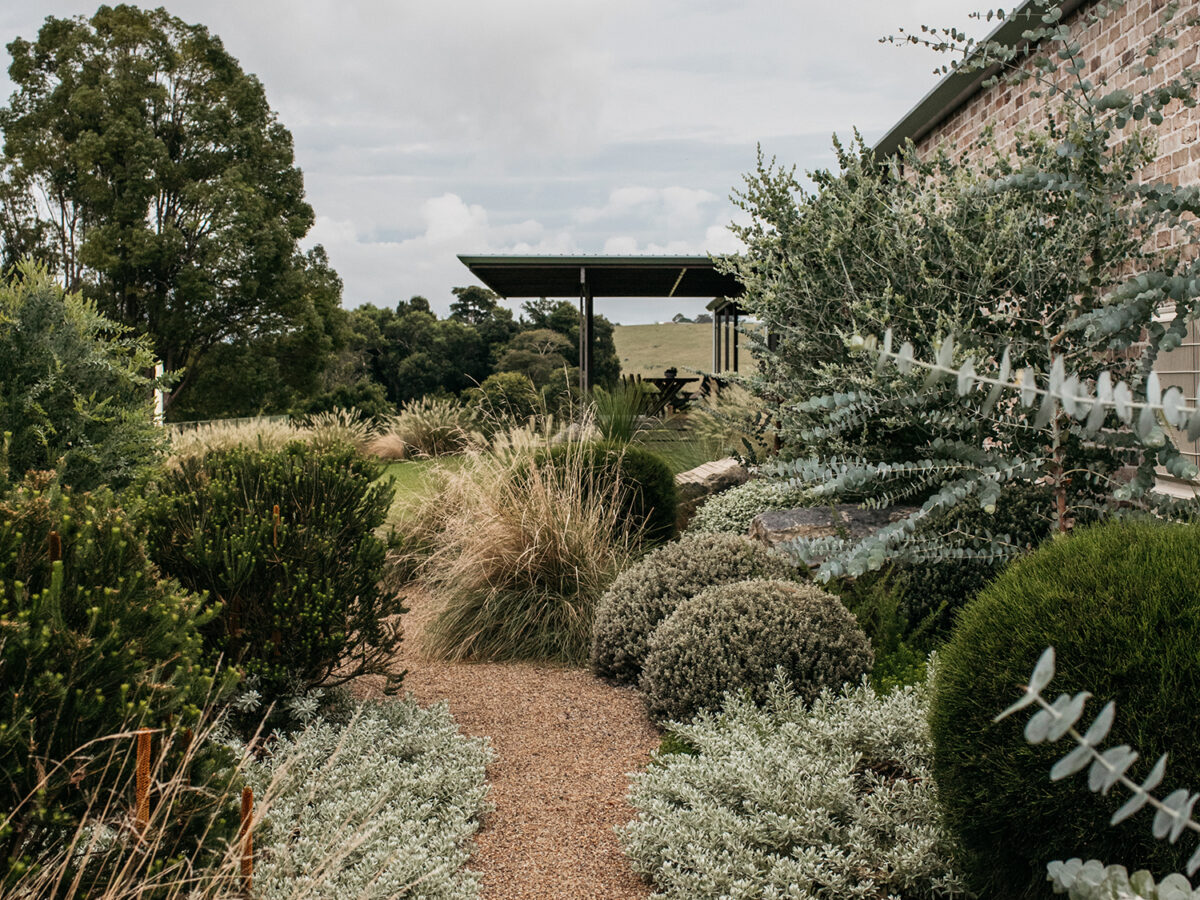The outdoor image showcases a beautifully landscaped garden path primarily composed of beige pebbles interspersed with small black and white stones. This curving pathway extends from the middle bottom and winds upward and to the left, bordered by meticulously maintained bushes in various shades of green, from dark to light, as well as some grassy brown shrubs. To the right, some of these bushes are pruned into perfect circles, demonstrating expert gardening skills. In the background sits a gazebo with a picnic bench under its large brown roof, offering a serene resting spot. On the left, a large tree adds to the garden's lush atmosphere, while a red brick wall stands prominently on the right. The sky above is cloudy, casting a slightly darker tone over the daytime scene, contributing to the overall tranquil and earthy ambiance reminiscent of a well-tended desert garden.